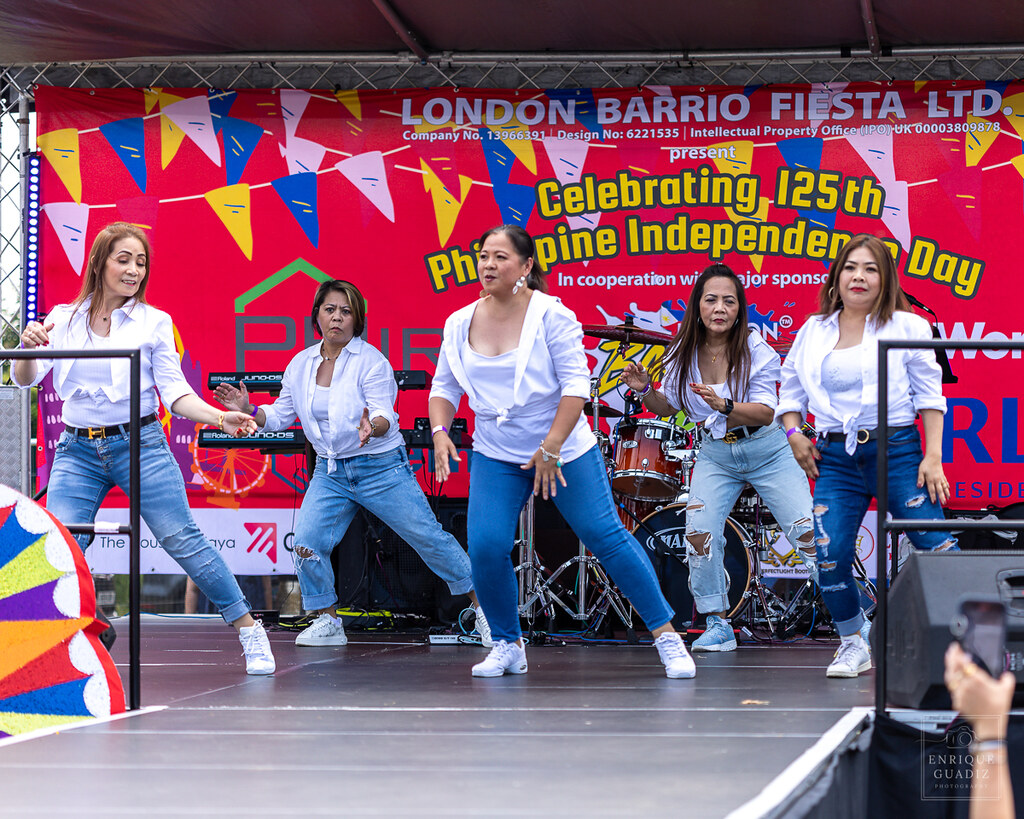This vibrant outdoor photograph showcases a lively scene at the London Barrio Fiesta Limited event, celebrating the 125th Philippine Independence Day. A group of five Asian women, likely Filipino, are captured in the midst of a dance performance on a gray stage with white borders. Each dancer is dressed in matching white shirts, denim jeans, and white sneakers, adding a cohesive aesthetic to their synchronized routine. 

The backdrop is dominated by a striking red banner adorned with colorful triangular flags in yellow, blue, and purple. The banner prominently displays text in white and yellow, reading "London Barrio Fiesta Limited presents celebrating 125th Philippine Independence Day." Additionally, there are design numbers 13966191 and 6221535, and an Intellectual Property Office watermark number 4038098278, hinting at image protection.

In the lower right-hand corner, an arm holding a camera is visible, indicating the presence of an engaged audience capturing the festive moment. On the stage, instruments including a drum set and keyboard suggest that the event features various performances. A touch of additional color is provided by color wheels positioned to the left side of the stage.